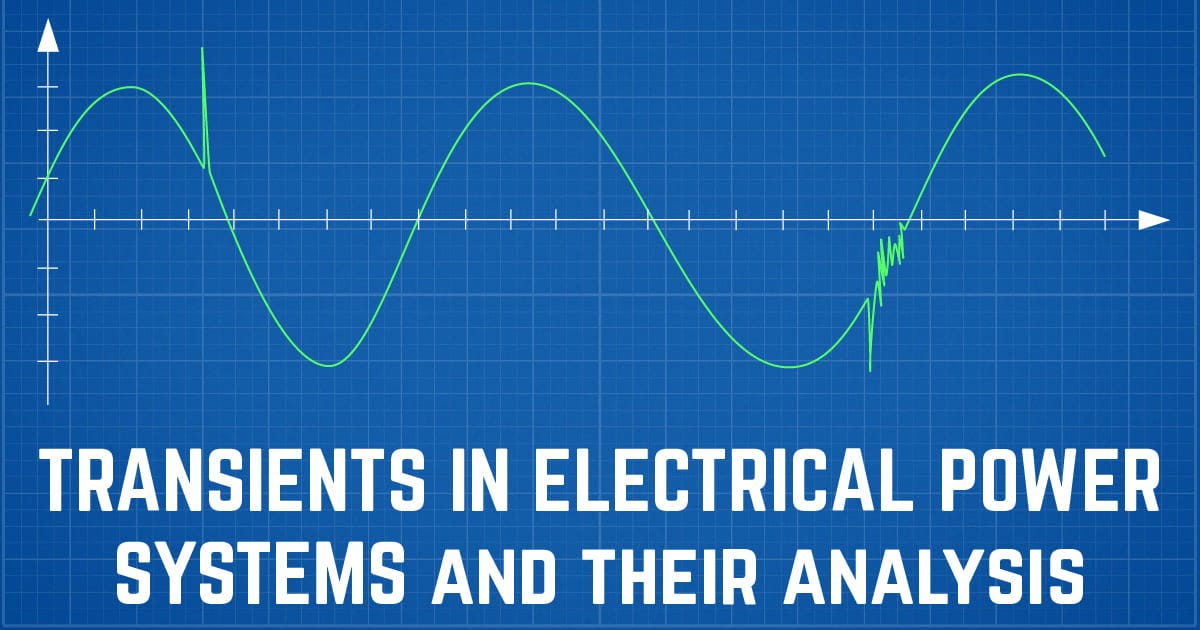The image showcases a detailed graph titled "Transients in Electrical Power Systems and Their Analysis" in white capital letters at the bottom of a horizontally rectangular blue background. The graph features white vertical and horizontal lines intersecting at regular intervals to form a grid. A bold white arrow points upwards along the y-axis, while another white arrow points to the right along the x-axis. The main feature of the graph is a green waveform line that oscillates up and down across the x-axis. It begins near the origin point, displaying dramatic variations, including two prominent spikes—an initial sharp uplift followed immediately by a drop, and later another sharp drop followed by an uplift. Towards the end, the waveform experiences a series of jagged fluctuations before returning to a more consistent pattern. The depiction captures the turbulent nature of electrical power transients, emphasizing periods of significant disturbance amidst a generally smooth wave.